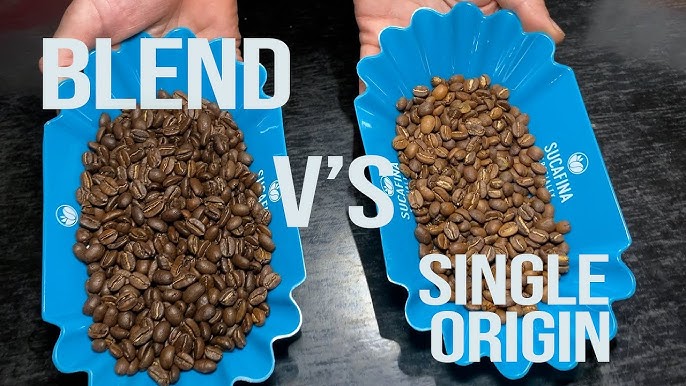The photograph features two blue bowls of coffee beans, each held by a hand against a black table. The bowl on the left contains dark brown beans labeled "BLEND," while the bowl on the right holds lighter brown beans labeled "SINGLE ORIGIN." Both bowls have a scalloped edging along the sides and partial white text visible inside spelling out "SUCAFINA" beneath a circular logo. The text on the image compares the two types of coffee beans, emphasizing their differences in color, likely indicating a difference in roast levels and origin. The hands holding the bowls are white, presenting these beans clearly for viewers.